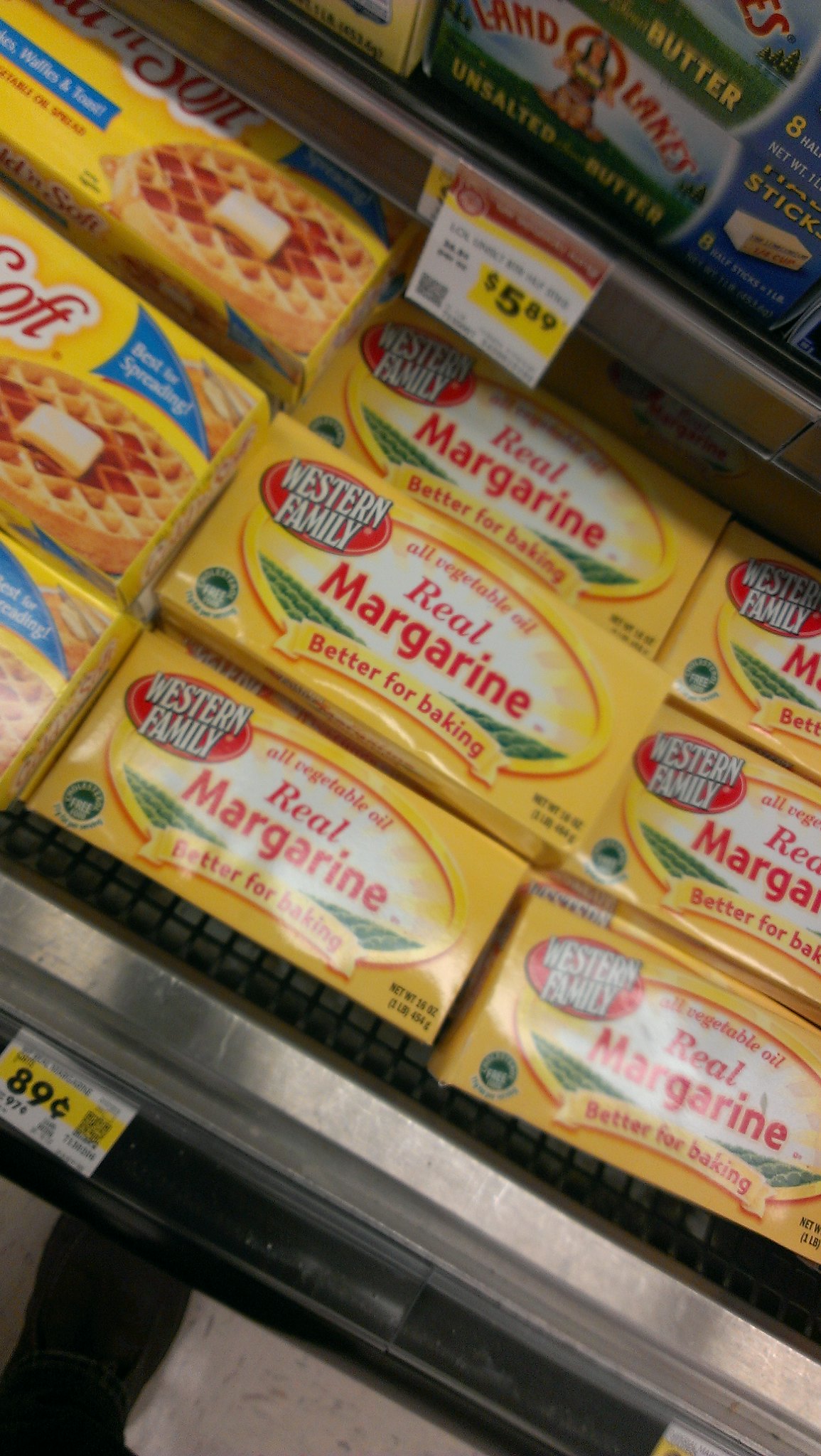In a detailed first-person perspective, the image showcases a supermarket's cold storage aisle, specifically the butter and margarine section. Captured from above with a phone tilted downwards, the photo includes the partial view of a man's right shoe and black pants on a polished marble floor with white and brown spots. The display shelf features prominently, segmented into two levels.

On the bottom shelf, vibrant yellow packages of Western Family Real Margarine are stacked, arranged in two columns and three rows, with a total of six visible packs. Each package features an orange circle in the upper left corner with "Western Family" in white writing, a central logo displaying "Real Margarine" in red font over a white background, and a picturesque valley scene with a "Better for Baking" banner below. The price tag for this margarine is highlighted in black text reading $0.89 on a yellow bar.

On the shelf above, packages of Land O'Lakes Unsalted Butter are visible. Distinguishable by their depiction of a Native American woman in a grassy landscape with a body of water and sky in the background, these packages include imagery of butter sticks on the right. The price tag here is larger, featuring a red border with white and yellow detailing, displaying the cost of 8 sticks at $5.99. 

Additionally, to the left of the Western Family margarine, there are more yellow butter packages showcasing an image of golden-brown waffles drizzled with syrup and topped with a melting butter slice. Adjacent to this arrangement, part of a white tiled floor with a silver-edged shelf is also visible, completing the detailed scene within the supermarket's dairy section.